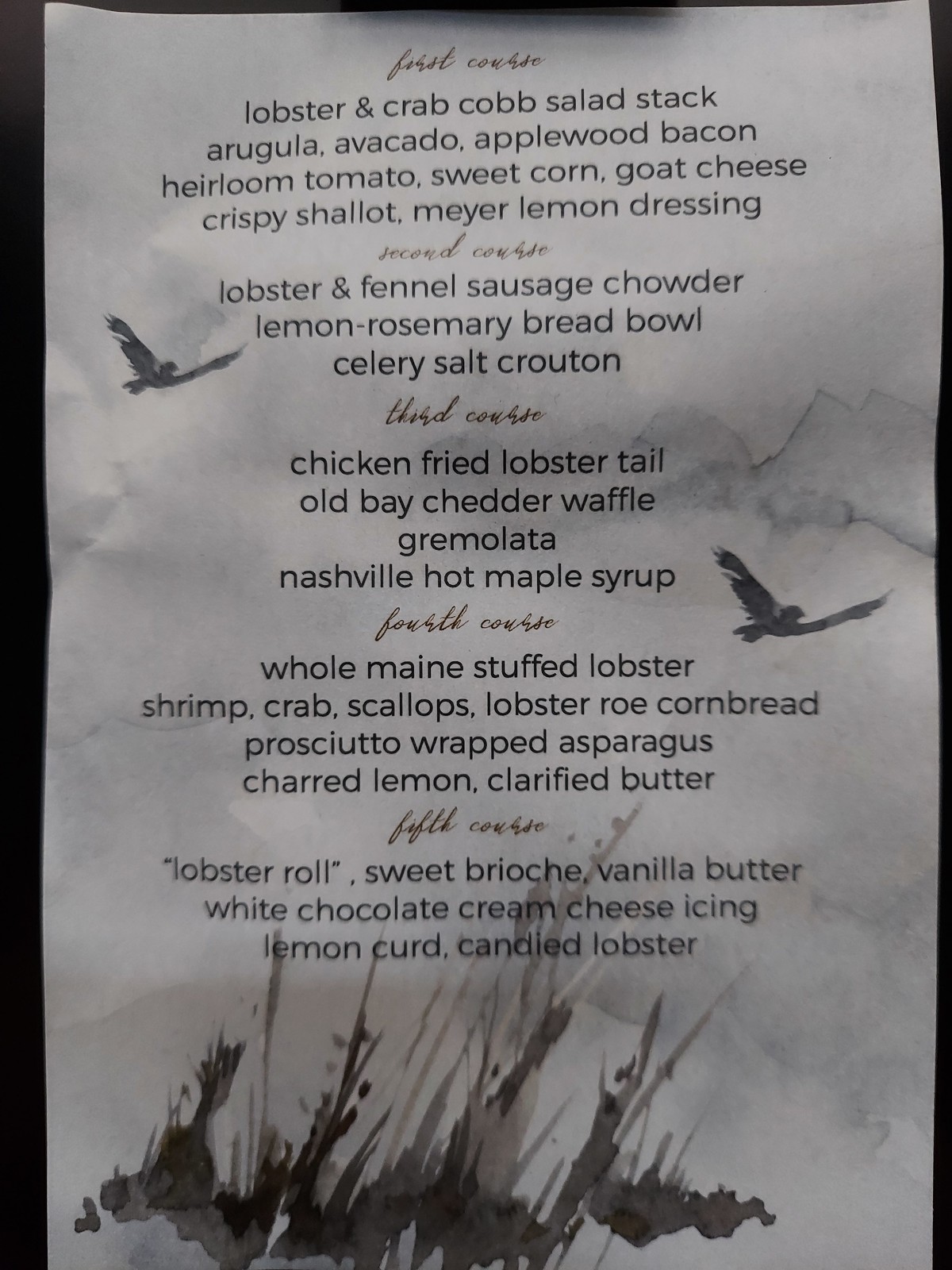This elegant menu is artistically designed to resemble a traditional Chinese painting, featuring serene mountain ranges nestled among the clouds. The paper itself is slightly crumpled, adding to the rustic and authentic vibe. At the bottom of this monochromatic menu, delicate watercolor brushstrokes depict grasses and little bushes, while a few birds soar gracefully in the sky above.

The menu is divided into five sections, each depicting a different course, all meticulously handwritten. 

**First Course:** 
- Lobster and Crab Cobb Salad Stack
  - Ingredients: Avocado (misspelled on the menu), Applewood Bacon, Heirloom Tomato, Sweet Corn, Goat Cheese, Crispy Shallot, Meyer Lemon Dressing.

**Second Course:** 
- Lobster and Fennel Sausage Chowder
  - Accompaniments: Lemon Rosemary Bread Bowl, Celery Salt Crouton.

Each course features a detailed list of ingredients, suggesting a unique and carefully curated culinary experience. The final course intriguingly includes a "lobster roll" served on sweet brioche with vanilla butter, topped with white chocolate and cream cheese icing, blending traditional flavors with an innovative twist. 

Overall, this menu not only promises a gastronomic delight but also invites you into a visual journey reminiscent of classic Chinese artwork.